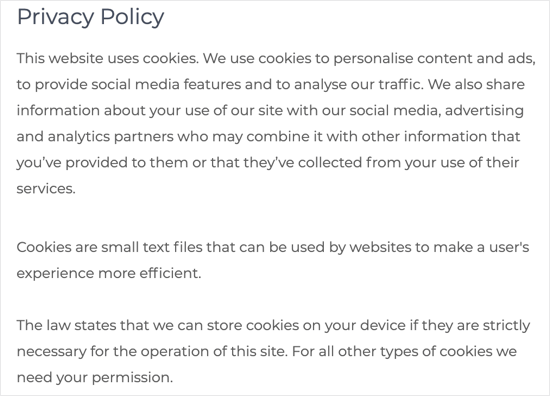This image showcases a section of a website's privacy policy in a visually distinct manner. The privacy policy text, written in bold black print for emphasis, is neatly enclosed within a light gray, rectangular border that helps to separate it from the rest of the page. The policy states that the website uses cookies for various purposes, including personalizing content and advertisements, providing social media features, and analyzing traffic. It notes that information about the user's interaction with the site is shared with social media, advertising, and analytics partners, who may combine it with other data collected from the user. By law, cookies that are essential for the website's operation can be stored on the user’s device without consent, but permission is required for all other types of cookies. The background surrounding this policy text is completely wiped clean, ensuring that the focus remains on the privacy information.